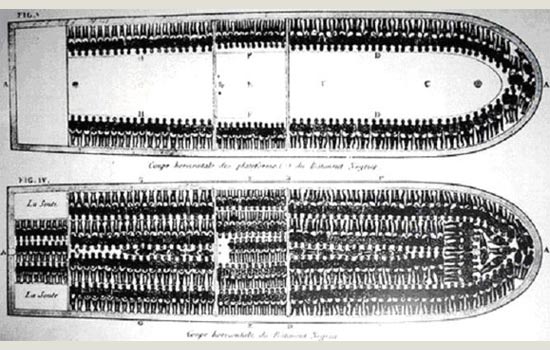This is a black-and-white, horizontally aligned rectangular image that appears to be a historic illustration showing the interior layout of a slave ship. The image has a beige border at the top and bottom, but no borders on the sides, set against a whitish-gray background. The main elements of the illustration are two elongated, rounded shapes resembling the hull cross-section of a ship, each divided into multiple sections.

The upper shape is shaded white with faint black lines outlining small, indistinct human figures, suggesting these are crowded compartments. There is cursive writing underneath this shape, but it is too small and faded to decipher clearly. 

The lower shape mirrors the upper one but is more detailed, with the left vertical rectangle featuring two white horizontal sections, one at the top and one at the bottom, each containing small black human figures, which likely represent enslaved Africans. The rest of this lower shape is similarly filled with tiny black and white figures, indicating the densely packed slaves within the ship. Visible along the top left corner of the image, there appears to be a figure number, potentially "Figure 3," and small cursive writing which seems to include French words, possibly indicating the origin of this diagram. The word "Congo" can be discerned between the two rounded shapes, further substantiating the historical context.